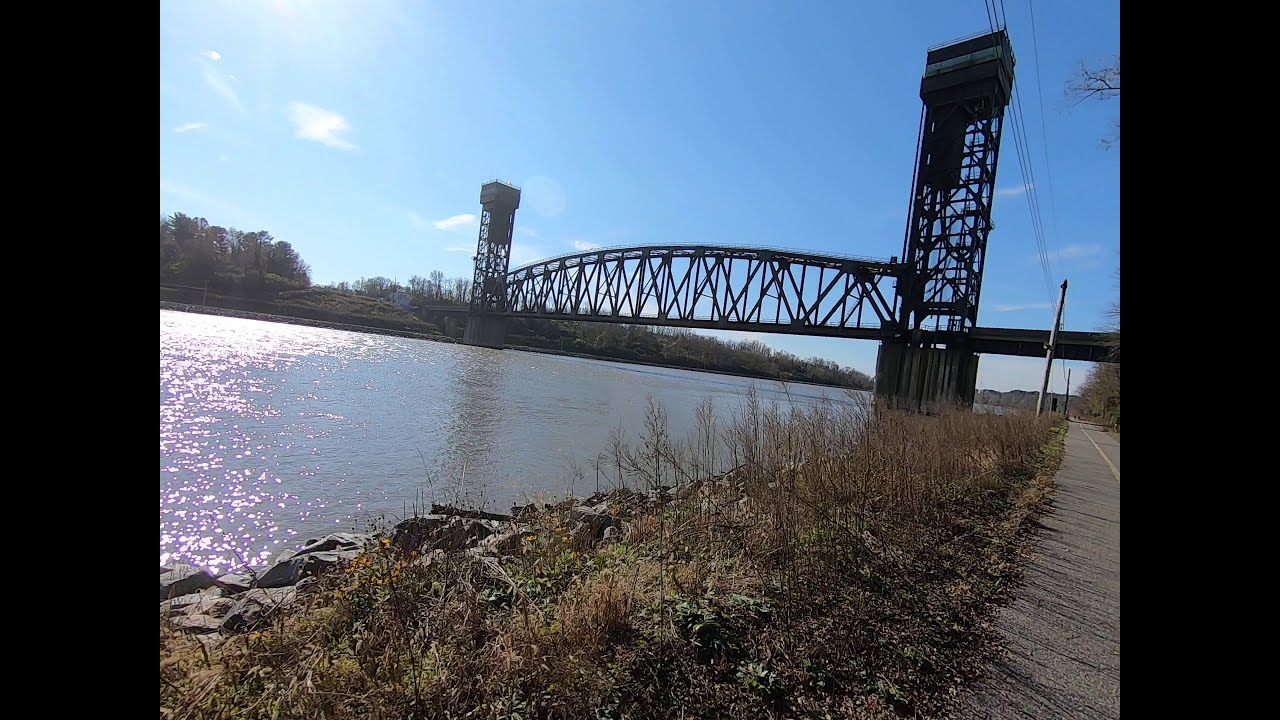This horizontal photograph, framed by wide black borders on either side, captures a river scene dominated by a large suspension bridge. The bridge features two very tall towers that descend into the muddy brown river, with the structure extending symmetrically from these central towers to the land on either side. The foreground is mostly barren, with dead weeds, rocks, and bare dirt lining the riverbank. On the right side, there is an old, narrow walking trail made of macadam that follows the shoreline, allowing pedestrians to walk along the river and beneath the bridge. The opposite riverbank is lined with trees providing a contrast to the sparse foreground. The sky above is mostly clear with a few clouds, and the overall scene is devoid of people or animals, contributing to a quiet, almost desolate atmosphere. Small details such as a twig or branch intruding from the upper right add an extra layer of natural texture to the image. Overall, the scene appears industrial and somewhat aged, giving it a character of its own.